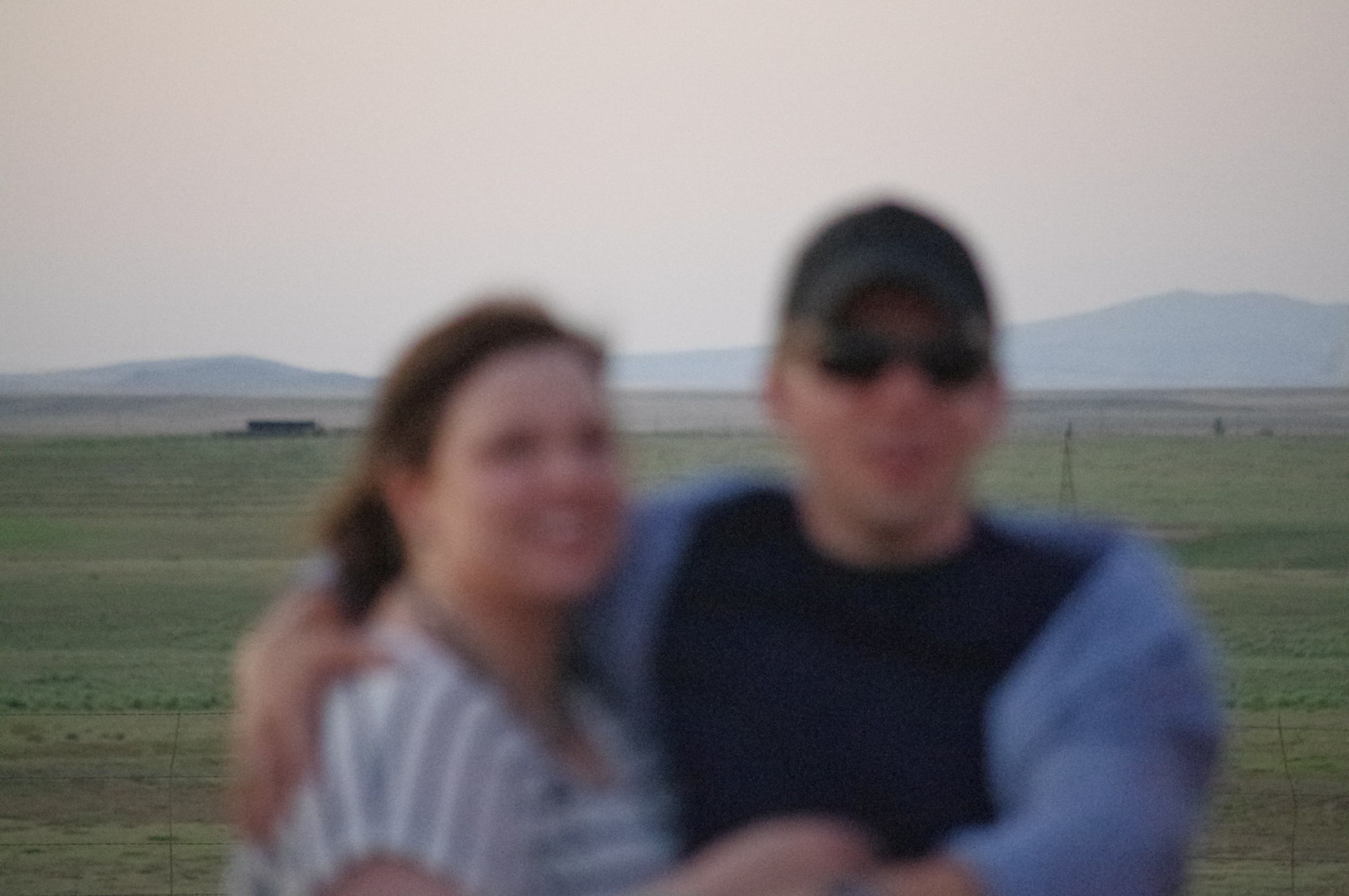In the photograph, two individuals are standing in the foreground, partially embracing, though the image captures them in a blurry manner, making their features difficult to discern. The background, in contrast, is more sharply defined, presenting a serene scene with a gradient sky transitioning from gray to a pinkish hue, and blue-gray mountains that span the horizon, rising slightly higher on the right side. Below the mountains, a strip of grayish-tan fields gives way to lush green fields, all extending horizontally behind the couple.

In the foreground on the left stands a woman with brown hair pulled back into a ponytail. She is dressed in a short-sleeved, striped blouse, possibly in gray and white, and she wears a faint smile, her facial details blurred. To her right is a man with light skin, dressed in a dark t-shirt, perhaps black or navy blue, and a matching dark blue baseball cap coupled with dark sunglasses. He seems to be wearing a light blue, sweatshirt-like jacket over his shirt. His right arm is wrapped around the woman, holding her close, and he too has a slight smile, though equally indistinct due to the blur. Despite the unclear details of their faces, the couple emanates happiness as they pose against the scenic backdrop.